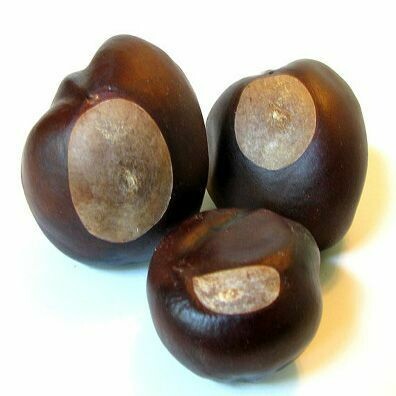This image features three dark brown, spherical nuts, each with a distinctive light brown splotch on them, suggesting characteristics of either chestnuts or macadamia nuts. The nuts are arranged in an upside-down triangular formation, with the largest on the upper left, the medium-sized on the upper right, and the smallest at the bottom center. They are set against a clean, white background, with shadows clearly visible behind them, providing an unobstructed view of their details. Their arrangement and the professional quality of the photograph hint that it might be intended for educational purposes, showcasing the nuts in their unshelled form.